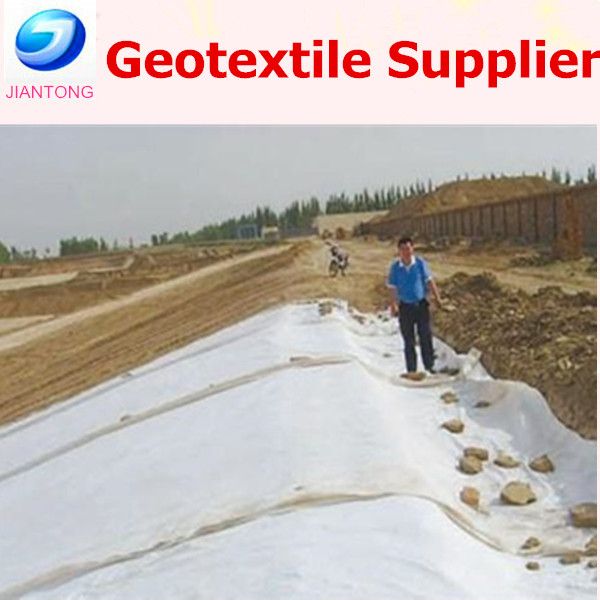The advertisement for Jiantong, a geotextile supplier, features a prominently placed banner photograph. The top of the banner displays the company's name "Jiantong" and their logo—a blue circle with the bottom part of a "G" extending in white. The red text above the logo reads "Geotextile Supplier." The image itself appears to be set in a rock quarry or a similar outdoor environment, illustrating a practical application of the geotextile product. In the foreground, a white geotextile sheet stretches down a slight slope, with rocks placed on top to secure it. A person, dressed in black pants and a blue collared shirt with a white collar, stands on the sheet within a ditch. In the background, a bicycle rests near a fence, with a hillside and pine trees completing the scene. The overall photograph resonates with rugged, natural tones of brown and green, though it is somewhat blurry and evokes a desolate, utilitarian atmosphere.